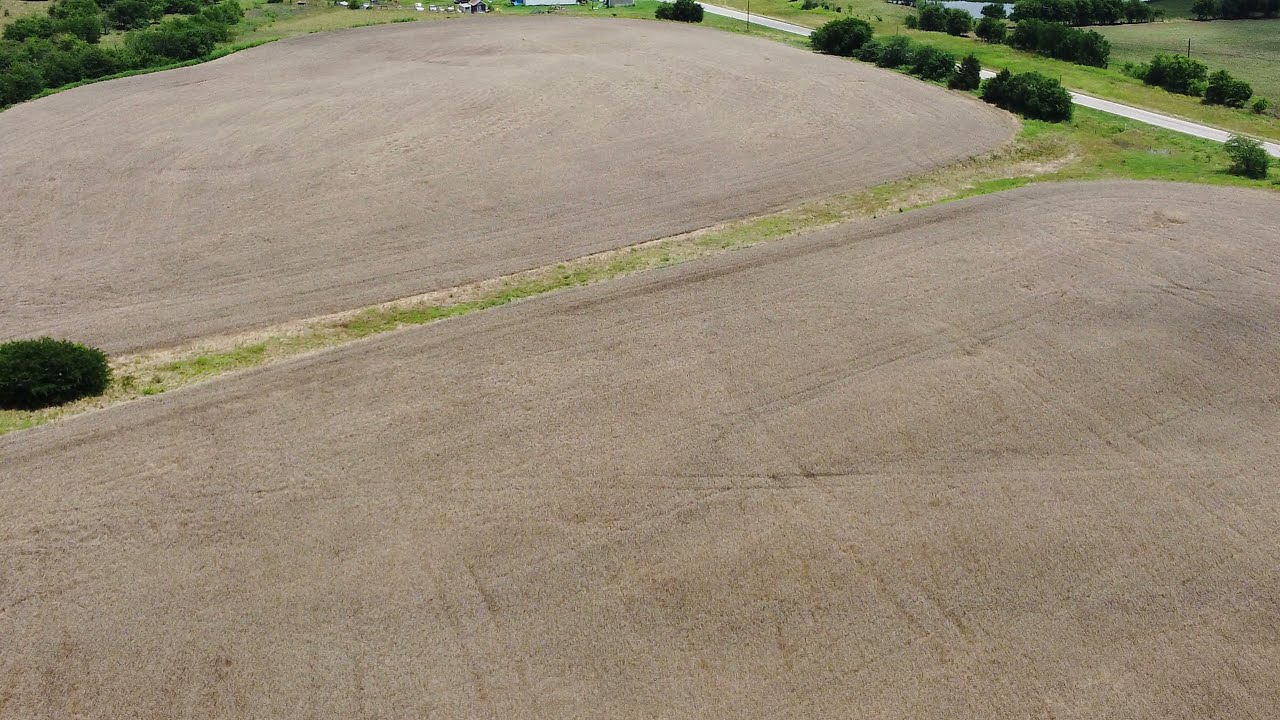The outdoor countryside scene is dominated by two expansive, plowed fields, devoid of grass, showing raw, flat dirt. The fields, one located at the bottom right and the other at the upper left, are bisected by a narrow, patchy strip of land still showing remnants of grass and housing a lone bush. The freshly plowed soil in both sections displays visible markings and uneven tractor treads, suggesting recent equipment activity but no seed sowing. Green shrubbery lines the upper left and right-hand corners, with a small, thin road meandering behind the shrubbery on the right, disappearing towards the horizon. The edges of the fields appear slightly rounded, resembling a large, deserted parking lot. In the distant background, on the upper left, there are additional bushes, a patch of grass, a hint of water, and possibly a few houses, indicating a rural residential area.